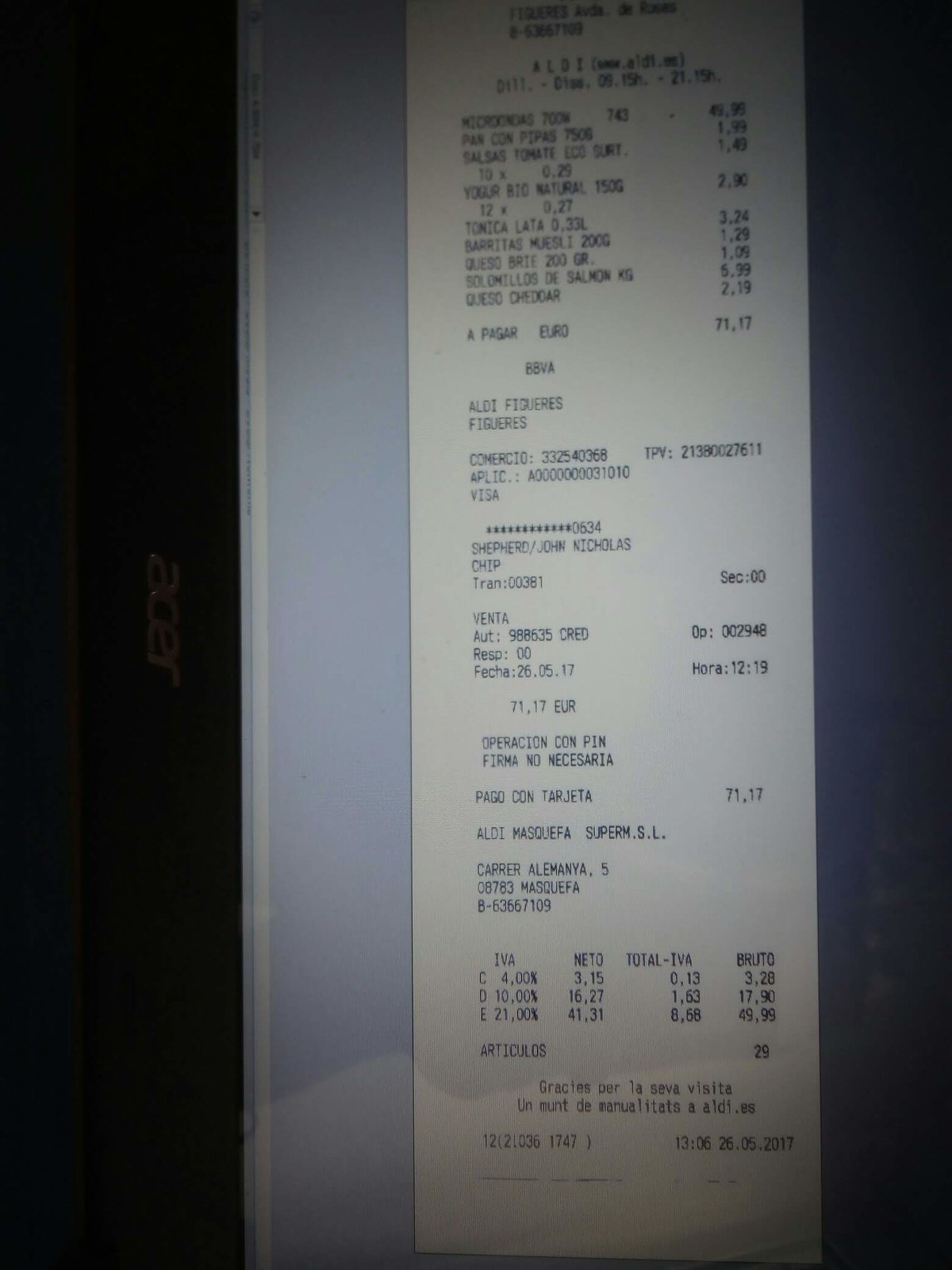This image is a photograph of a grocery receipt from Aldi, displayed on an Acer laptop screen. The receipt, written in Spanish, totals €71.17. It features items such as queso cheddar, yogurt, muesli, pasta, cheese, and salmon. The laptop, oriented vertically to display the lengthy receipt, shows it photographed in a program with a gray background and navigation buttons along the left bar. Key details on the receipt include a payment via Visa, a cashier named John Nicholas, and a timestamp of 1:06 PM on May 26, 2017. Near the bottom of the receipt, the word "gracias" is visible, indicating a courteous sign-off.